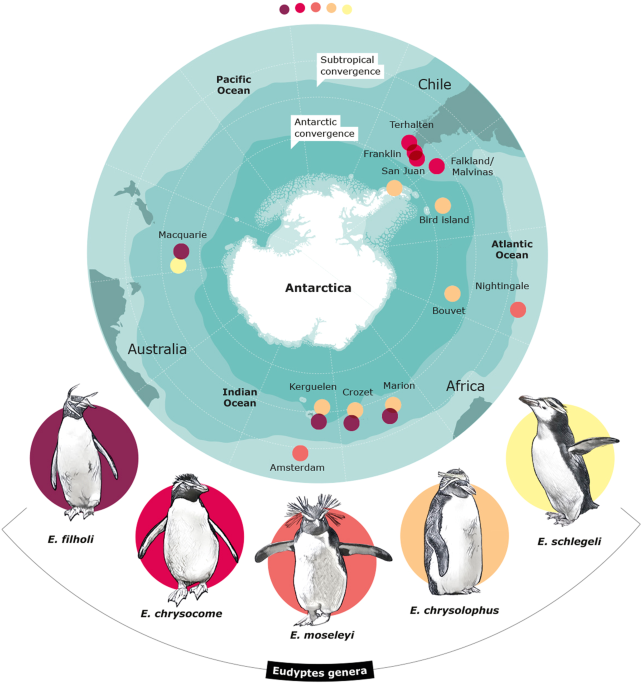This image is a detailed world map, prominently featuring Antarctica in the center, which illustrates the distribution of various species of penguins across the globe. It highlights key regions like Chile, Australia, and Africa, and marks the major oceans: the Pacific, Atlantic, and Indian. The map uses colored dots to indicate the habitats of five distinct species of penguins. Each species is represented by a specific color: purplish-red for E. philholi, red for E. chrysocome, pinkish for E. moseley, orange for E. chrysolophus, and yellow for P. adeliae. Alongside the map, there are images of each penguin species, showcasing their unique physical characteristics, such as variations in feather patterns and coloration—some with crests of feathers on their heads and others with different black-and-white patterns. These visual and color-coded elements comprehensively reveal where each species can be found throughout the Antarctic region and the surrounding oceans, offering a clear depiction of their global habitats.